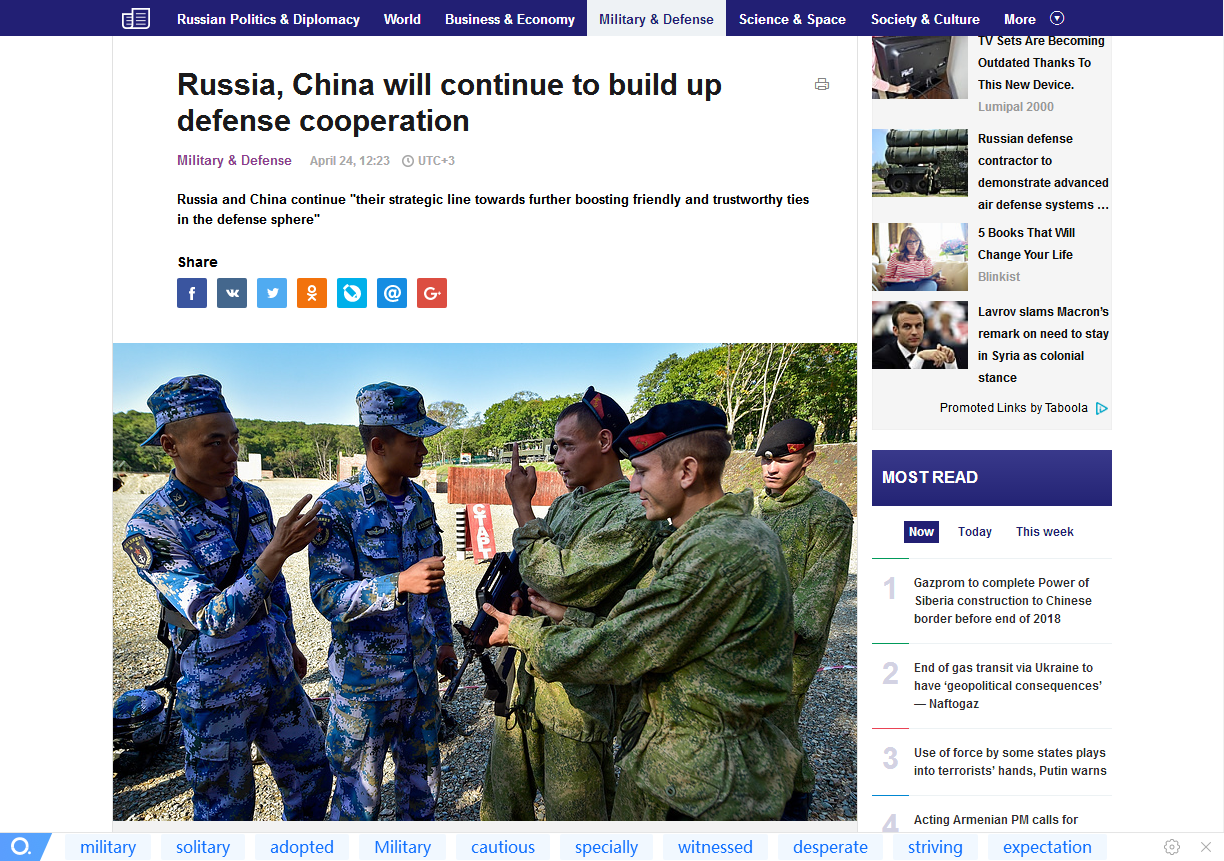A screenshot from a news website highlights an article titled "Russia, China Will Continue to Build Up Defense Cooperation." The article underscores the ongoing commitment between Russia and China to enhance their "strategic line towards further boosting friendly and trustworthy ties in the defense sphere." The image shows military personnel from both nations engaged in conversation, symbolizing the close defense relations they share. Surrounding the article, the website features various navigational elements: icons to share the article via Facebook, Twitter, and Google Plus, and a menu strip at the top with categories such as Russian Politics and Diplomacy, World, Business and Economy, Military and Defense, Science and Space, and Society and Culture, along with a pull-down menu for more topics. Down the right side, thumbnails link to other articles, including a piece titled "Five Books That Will Change Your Life." Below, there is a section highlighting the most read news articles.